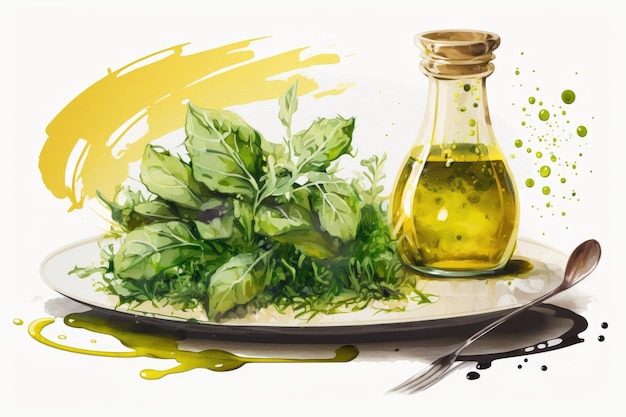The watercolor painting depicts a still life scene centered on a large, round, ceramic-looking white plate filled with a pile of fresh, green leafy greens, possibly basil or spinach. To the right of the plate is a small, glass jar with a cork closure, tapering towards the top and filled with what appears to be olive oil. Adjacent to the plate, there is a unique utensil with a fork on one end and a spoon on the other. Beneath the plate, on the left side, a swirl or splash of olive oil is visible, while on the right side, the black swirls and drippings suggest the presence of balsamic vinegar. In the background, the artist has added a few yellowish paint strokes and scattered green dots, enhancing the composition with a sense of depth and texture. The entire illustration is framed within a rectangular white border, capturing the essence of a simple yet elegant culinary setting.